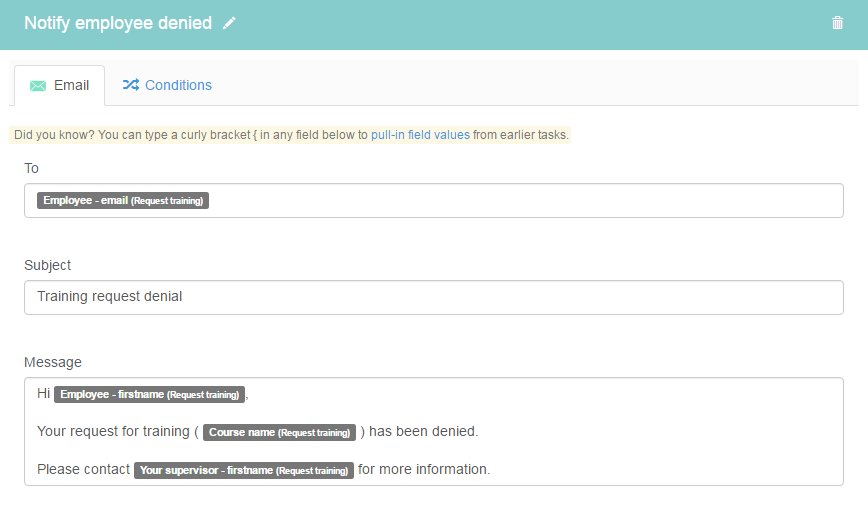In this image, we see a screenshot of a form used to notify employees about denied training requests. At the very top, there is a section labeled "Notify Employees Denied." In the top-right corner, there is an icon resembling a trash or delete button. Below the email header, there is a message stating, "Did you know? You can type a curly bracket {} in any field below to pull in field values from earlier tasks."

The form includes a field labeled "To," where it shows a placeholder text "employee or email," followed by an example of using curly brackets to auto-fill data: "{request_training}." 

The "Subject" field contains "Training Request Denial." The "Message" field is composed of several parts, dynamically pulling in values using curly brackets. The message begins with "Hi {employee_first_name}," followed by "{request_training}," and then continues with, "Your request for training {course_name} has been denied. Please contact your supervisor {supervisor_name} for more information."